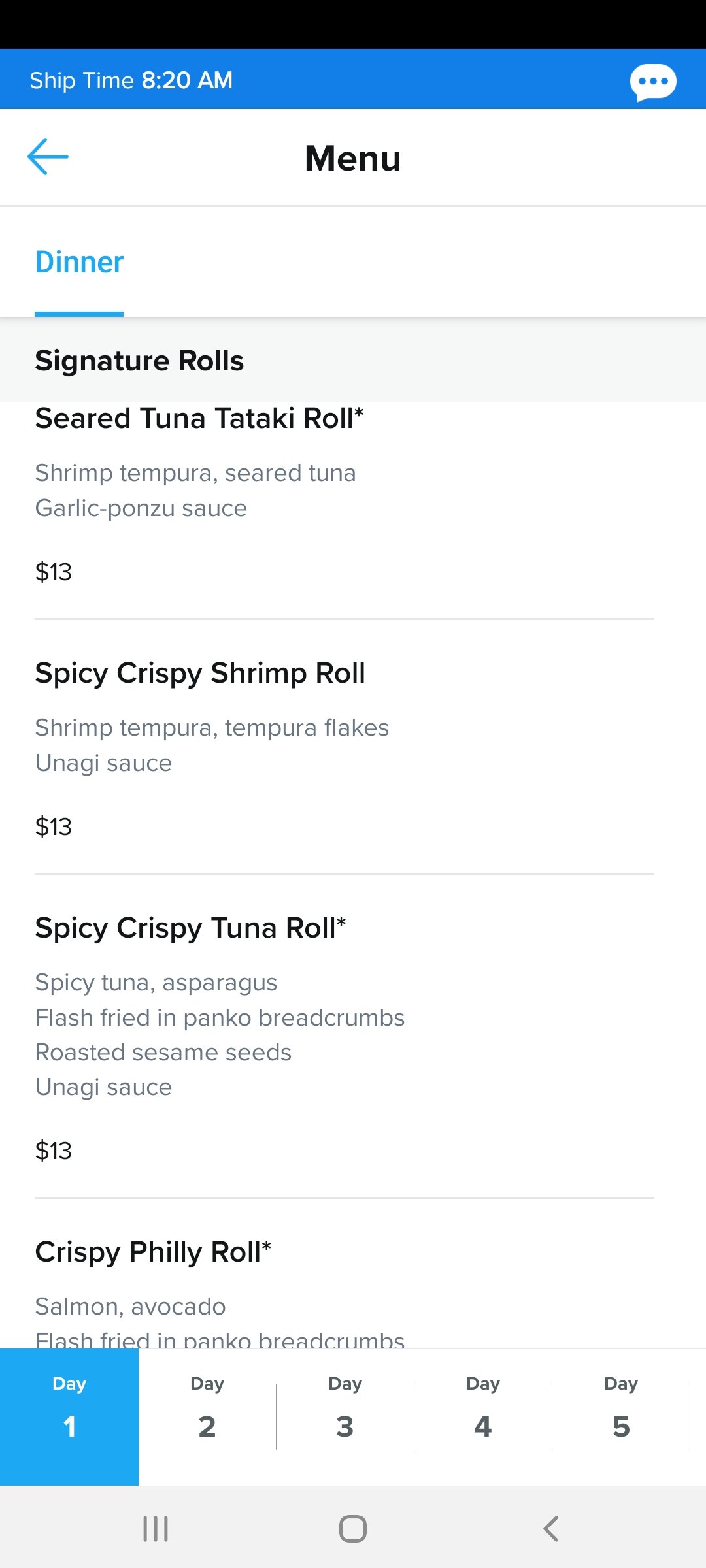The image depicts a food delivery app, possibly Uber Eats, displayed on a smartphone or tablet screen. At the very top, a black bar stretches across the screen from left to right. Directly beneath it, a dark blue strip also extends across the screen. In the top left corner of this dark blue strip, the text reads in white, "Ship time 8.20 am," while a messenger bubble icon rests on the far right.

Below these strips, a light blue back arrow points to the left. Bold, black text centered on the page announces "Menu." 

Underneath this, the section for "Dinner" is marked in blue on the left side. The user appears to be browsing the menu, though they have not made any selections yet. 

The menu itself has a light grey strip running horizontally across the screen, which is labeled "Signature Rolls" in black text. 

1. **Seared Tuna Tataki Roll**: Shrimp tempura, seared tuna, garlic ponzu sauce - $13. A faint grey line separates this item from the next.
2. **Spicy Crispy Shrimp Roll**: Shrimp tempura flakes, unagi sauce - $13. Another faint grey line follows.
3. **Spicy Crispy Tuna Roll** (marked with a star): Spicy tuna, asparagus, flash-fried in panko breadcrumbs, roasted sesame seeds, unagi sauce - $13. This is followed by yet another faint grey line.
4. **Crispy Philly Roll**: Salmon, avocado, flash-fried in panko breadcrumbs. The rest of the menu details are not visible.

At the bottom of the screen, a navigation bar displays day selections, starting with "Day 1" (currently highlighted in blue), followed by "Day 2," "Day 3," "Day 4," and "Day 5."